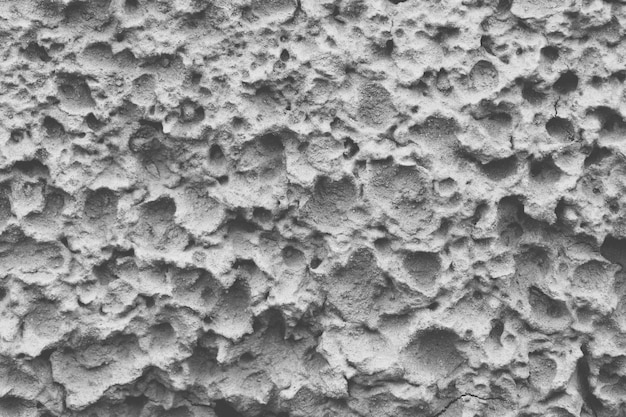This is a highly detailed close-up black, white, and gray photograph of an extremely textured surface. The material appears rough and jagged, featuring numerous small holes, pits, and valleys, evoking the appearance of pumice stone, hardened mud, or even a volcanic rock. The surface texture is deeply uneven, with shadows accentuating the dips and contours, resulting in a grayscale color palette with variations from light gray to dark gray. There are no signs of life or any other distinguishing features; it is solely the intricate texture of the material itself that fills the frame. The image consistently maintains this rugged structure throughout, and its true nature remains ambiguous, potentially resembling anything from organic matter to an extraterrestrial surface pockmarked by countless micro-collisions over time.